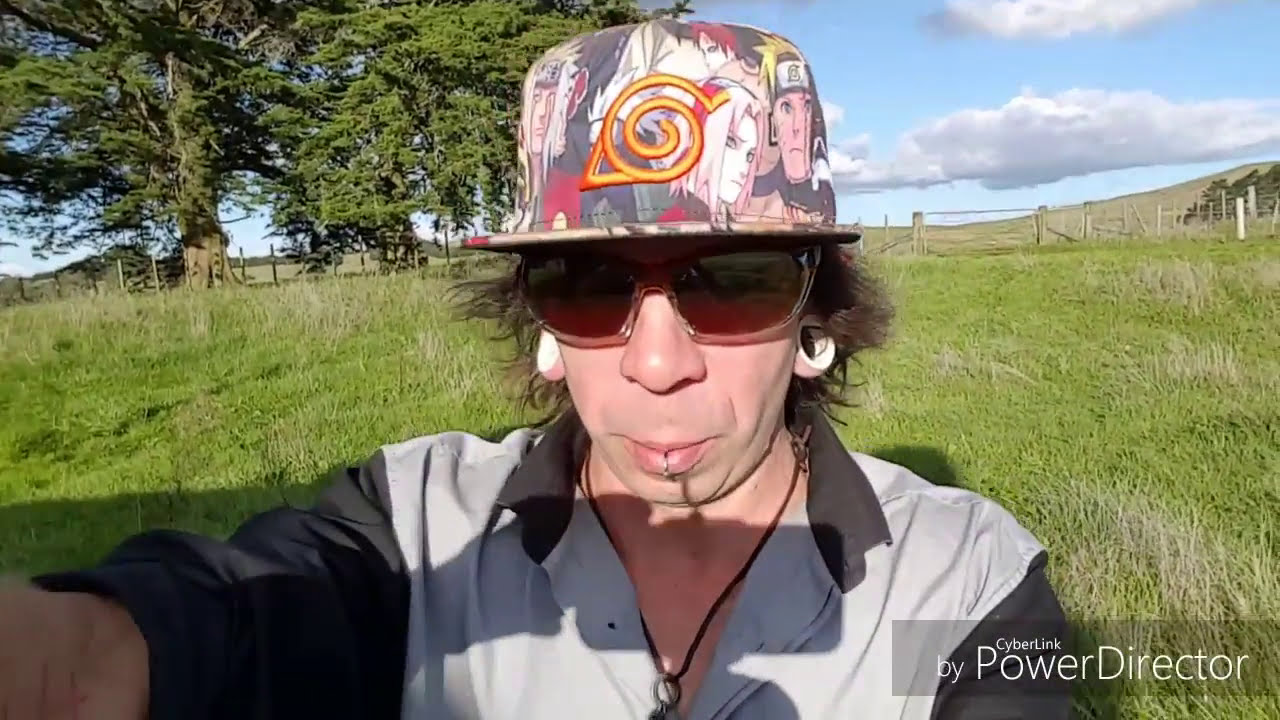In the image, a man positioned directly at the center captures attention with his hat adorned with various anime patterns and a swirl resembling a snail. He sports large red sunglasses and two significant hoop earrings inside his earlobes, with a lip ring dividing his lip. A black string necklace with a shell pendant hangs against his white button-down shirt with black sleeves. The man stands amidst a tall field of grass interspersed with hay, set against the backdrop of a blue sky punctuated by clouds and surrounded by a distant line of trees. The photo, appearing to be taken outdoors in the middle of the day, also features the text "CyberLink by PowerDirector" in the bottom right corner. The vivid colors in the image include shades of gray, tan, white, black, red, pink, green, and light blue.